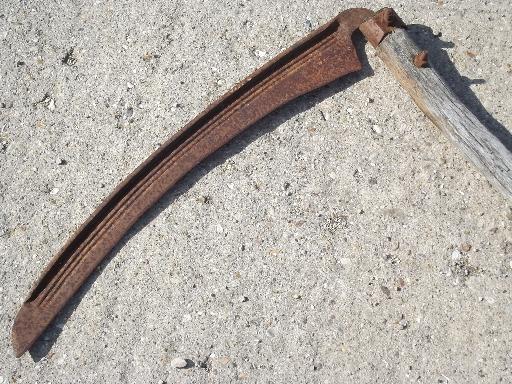The photograph captures a close-up of an ancient, rust-covered scythe, prominently displaying its severely oxidized metal blade. The blade is firmly fastened to a rough, aged wooden handle by two equally rusted nuts and bolts. The wooden handle, appearing gray and weathered, extends about six inches into the frame, showing signs of significant decay. The setting is an outdoor scene with the scythe lying on a coarse, unfinished concrete surface speckled with protruding stones and patches of dried vegetation, indicating a long period of exposure to the elements. Sunlight enhances the visibility of the tool's deterioration, emphasizing its long-abandoned state against the rough cement backdrop.